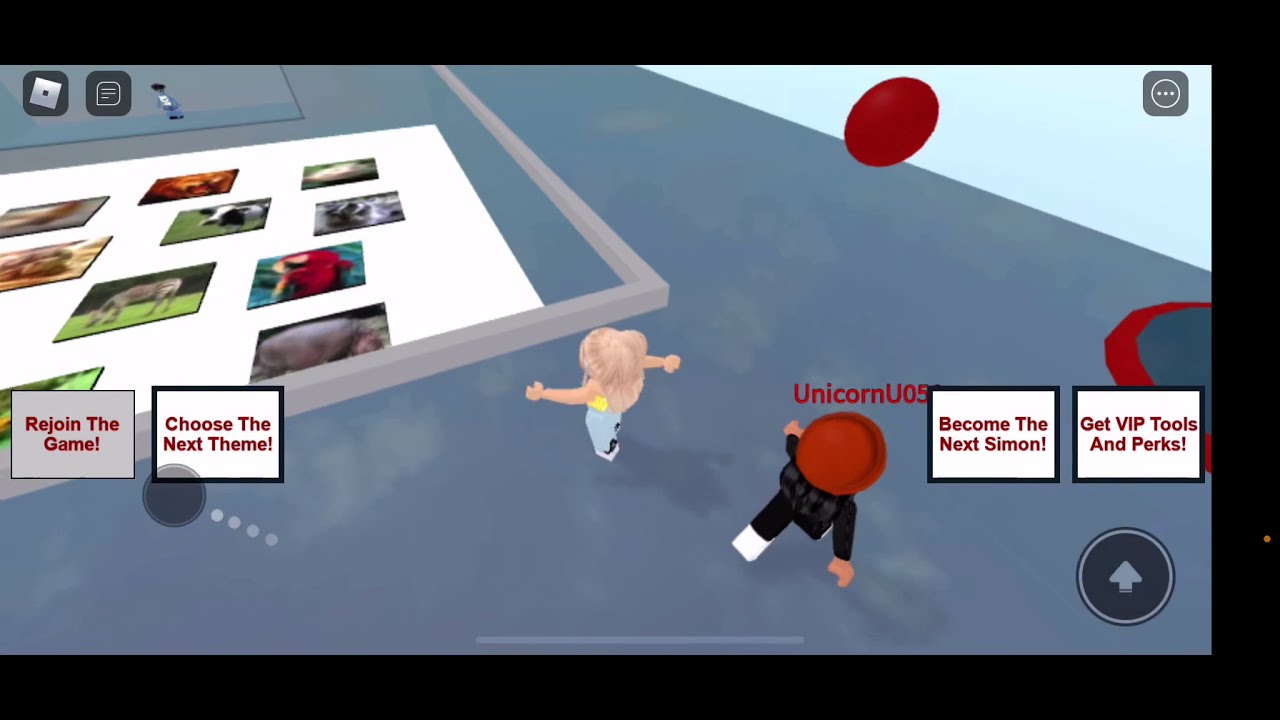This detailed screenshot from a video game features a flat, bluish-gray surface stretching towards a light blue sky in the top right corner. There, a prominent red oval is visible. Thick black borders frame the bottom, top, and right sides of the image; the left side is border-free. The central focus of the screenshot lies on two cartoonish video game characters: one with long blonde hair, a yellow shirt, and blue jeans, and the other in a black outfit topped with a red hat. Both characters face away from the viewer. 

The blonde character approaches an area featuring a collage of animal pictures on a white surface with a gray border, while the character in the black outfit seems to be moving towards a collection of letters and blocks. These blocks, placed two on the right and two on the left, bear the words: "become the next Simon", "get VIP tools and perks", "choose the next theme", and "rejoin the game". A distinctive black arrow encased in a circle points towards this text, which might imply interaction instructions. 

Additionally, several discs are scattered around, mirroring the one atop the character in black. The ground is a grayish hue, resembling watercolor or acrylic paint. To the left, the animal pictures suggest an interactive or thematic element in the game, indicating that the blonde character might be heading there to select the game's theme or engage with the environment.